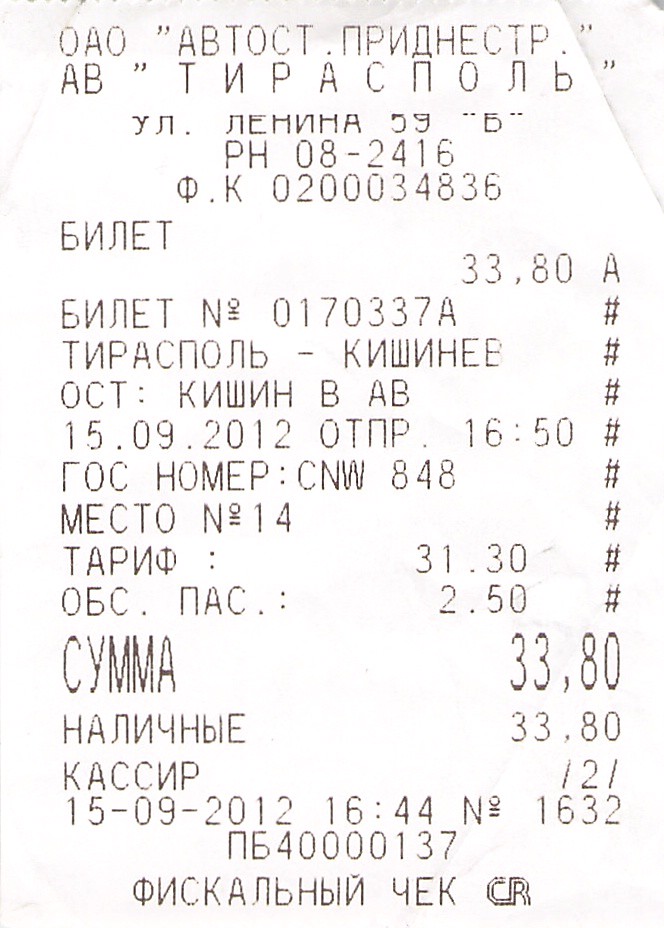This close-up image features a white receipt, primarily written in either Russian or Ukrainian. The text on the receipt is in black, covering almost the entire document from top to bottom. The total amount displayed is "33,80," with the date clearly marked as "15-09-2012 16:44." Although the background is predominantly white, there is a slight gray shading near the top edge of the receipt. No additional background elements are visible, focusing attention solely on the receipt's details.